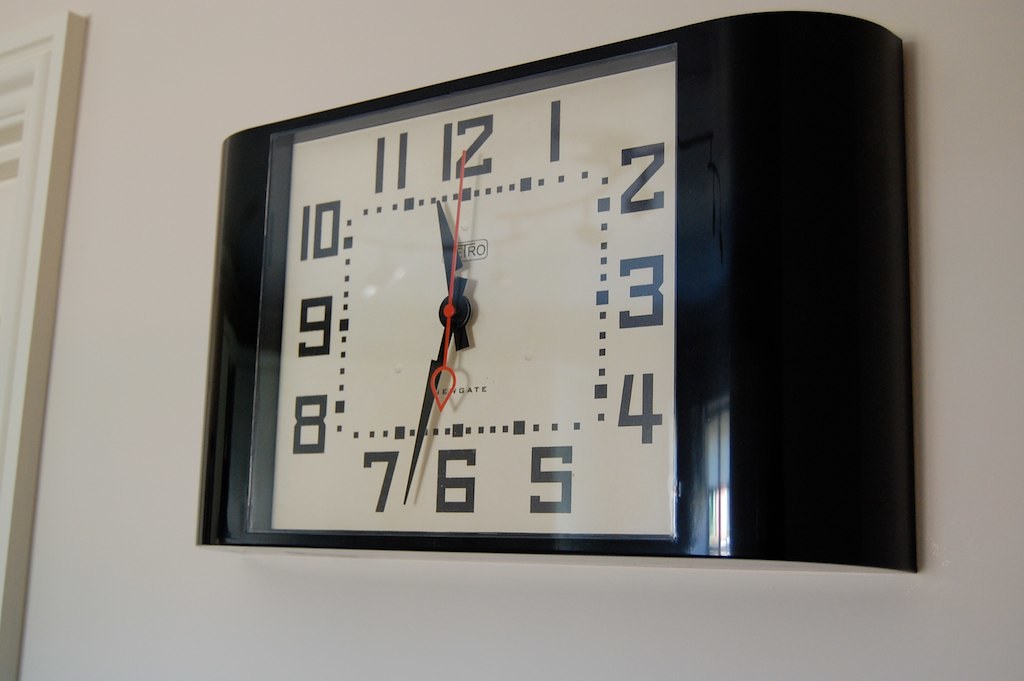A close-up image captures a rectangular clock with a sleek black frame, prominently displayed on a white wall. The camera, positioned to the right of the clock at eye level, tilts slightly to the bottom left, between 5 to 15 degrees, offering a unique angled perspective. The time on the clock reads 11:33. The clock face features standard numerals arranged around the rectangular frame, with 12, 11, and 1 at the top, 2, 3, and 4 on the right, 5, 6, and 7 at the bottom, and 8, 9, and 10 on the left. Surrounding the numerals, the hour marks are delineated by larger black squares, while the minute marks are represented by smaller black squares, adding a modern touch to the classic timepiece.